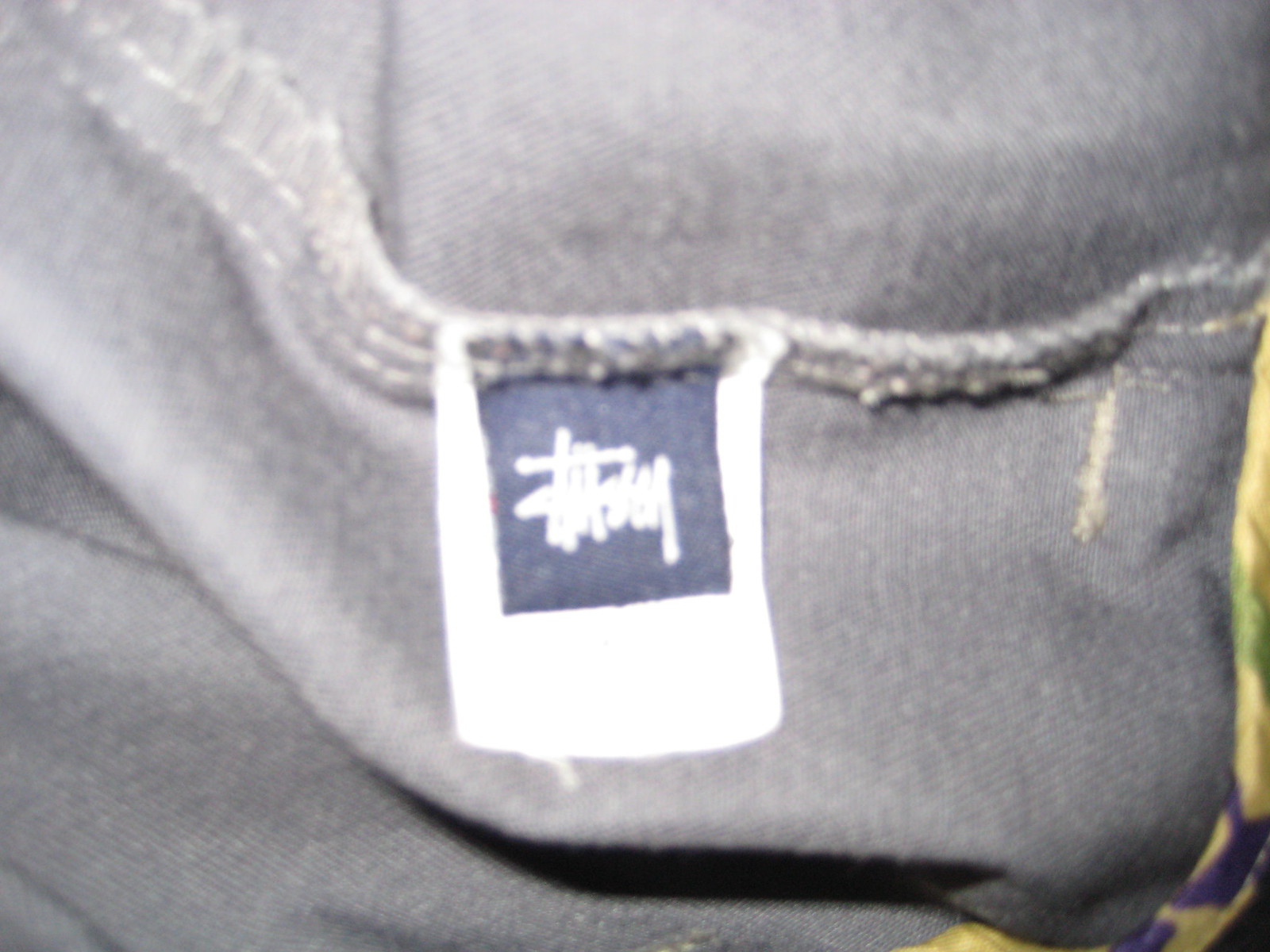Blurry image depicting a well-worn fabric piece. The fabric appears to be a dark shade, possibly bluish-black, accented with yellow or gold stitching. A prominent white tag is centrally positioned, though its details are unclear. Overlaying this white tag is a smaller, dark tag featuring white writing and a logo characteristic of the Stussy brand, though the logo is not fully legible. To the right, patches of yellow, green, and blue suggest the presence of another patterned fabric integrated into the garment.